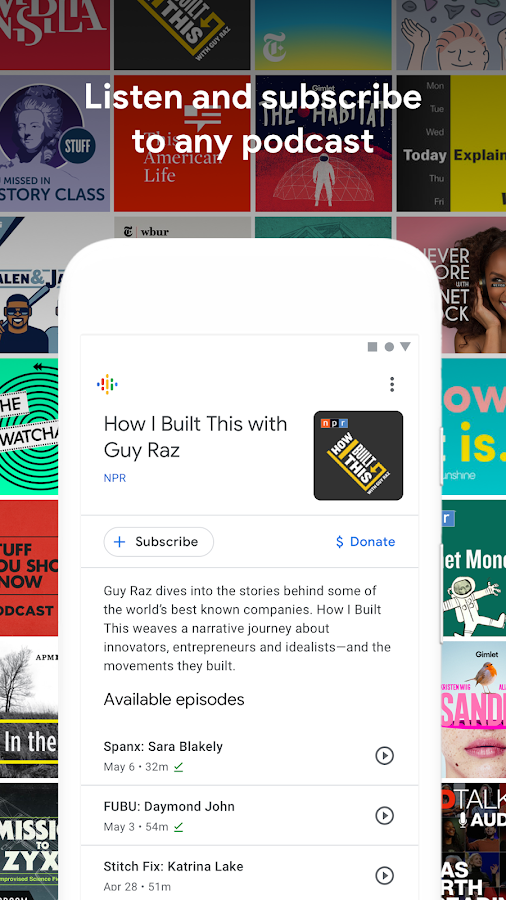This image is a screenshot taken from a mobile phone displaying a podcast app interface. The background showcases cover art for various podcasts, arranged in multiple rows of squares, each bearing the name of a different podcast. At the top of this background, a white font message reads: "Listen and subscribe to any podcast."

In the foreground, a white pop-up menu is prominently featured, focusing on a specific podcast. The title "How I Built This with Guy Raz" is written in black font, accompanied by its distinctive cover art—a creatively designed, rectangular graphic with the podcast's name.

Below the podcast title, there are two actionable buttons: a blue plus sign with the text "Subscribe" and a blue dollar sign labeled "Donate." Underneath these buttons, a detailed description of the podcast is provided. It reads: "Guy Raz dives into the stories behind some of the world's best known companies. 'How I Built This' weaves a narrative journey about innovators, entrepreneurs, and idealists, and the movements they've built."

Further down, three episodes are listed:
1. "Spanx with Sarah Blakely" – May 6 – 32 minutes
2. "FUBU with Daymond John" – 54 minutes